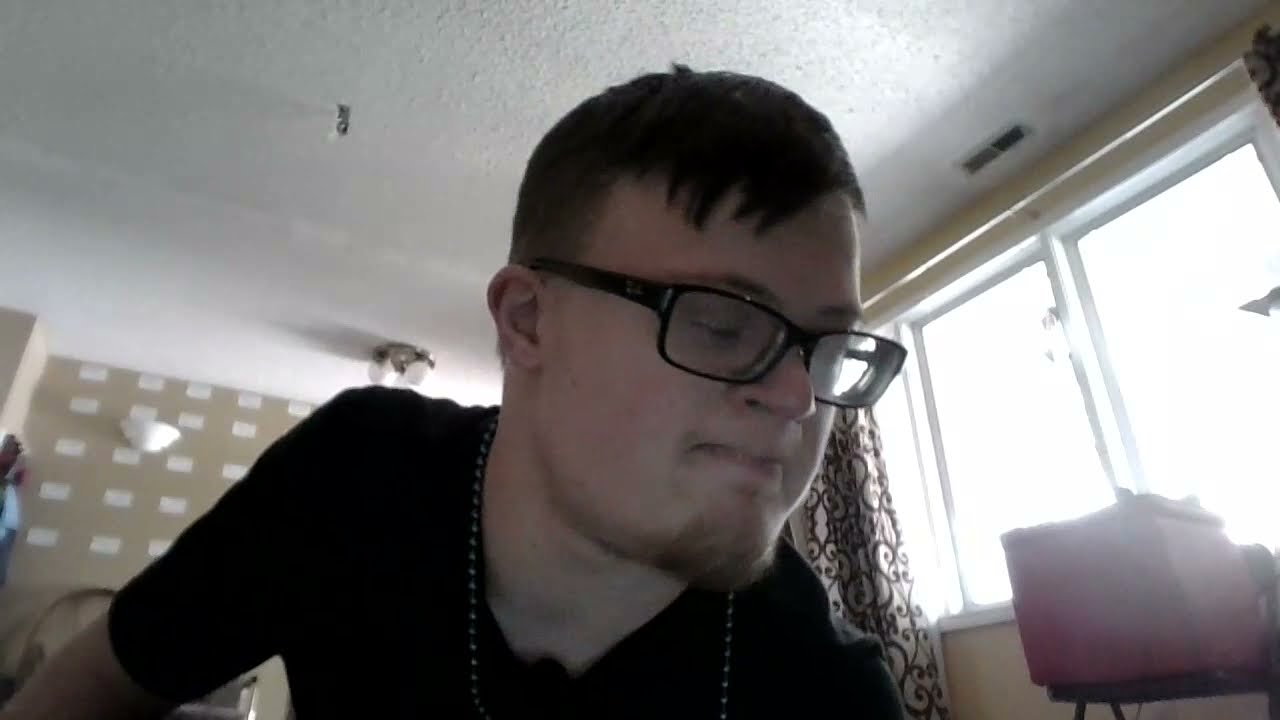This is an image of a man, likely in his 20s, captured from what appears to be a webcam or a self-taken photograph. The man is positioned slightly at an angle, looking down towards the right side of the image with his eyes closed, giving an impression of discomfort. He has short, dark brown hair, which is slightly balding, and a thin brown goatee that extends up to his ears, forming a light chin strap beard. He's wearing rectangular, thick-rimmed black glasses and a black beaded necklace, as well as a black long-sleeved shirt or t-shirt.

In the background, there are large windows emitting bright white light, making the room appear darker in comparison. Beige curtains with a brown curly pattern hang beside the window. A beige board with white Post-it notes or pieces of paper is also visible, alongside the ceiling vent. The room features contrasting elements with a tan wall covered with white squares, white ceiling, and a section of yellow wall on the right-hand side. The setting suggests he's in a bedroom or similar personal space.